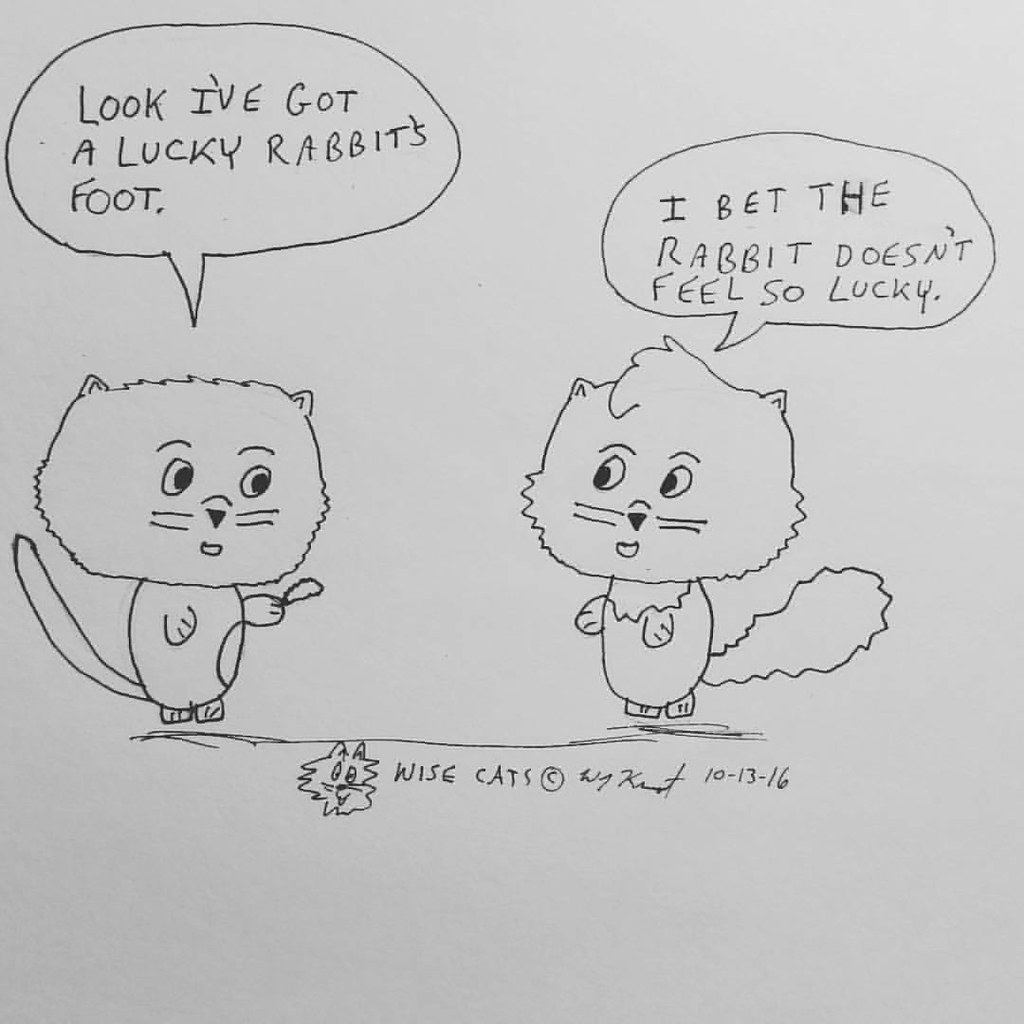This is a detailed photograph of a hand-drawn single-panel cartoon on white paper, created with black ink or pencil. The drawing features two cats standing on their hind legs, engaging in a conversation. The cat on the left, which has a long, thin tail and no tuft of fur on its head, appears more masculine and is holding up a rabbit's foot, saying, "Look, I've got a lucky rabbit's foot" in a speech bubble above its head. The cat on the right, characterized by a bushy tail and a tuft of fur atop its head, looks more feminine and responding with, "I bet the rabbit doesn't feel so lucky" in a speech bubble. Beneath the characters, there's a smaller drawing of a cat's head alongside the text "Wise Cats" with a copyright symbol. The signature of the author or illustrator, although unintelligible, is also present, accompanied by the date "10.13.16."